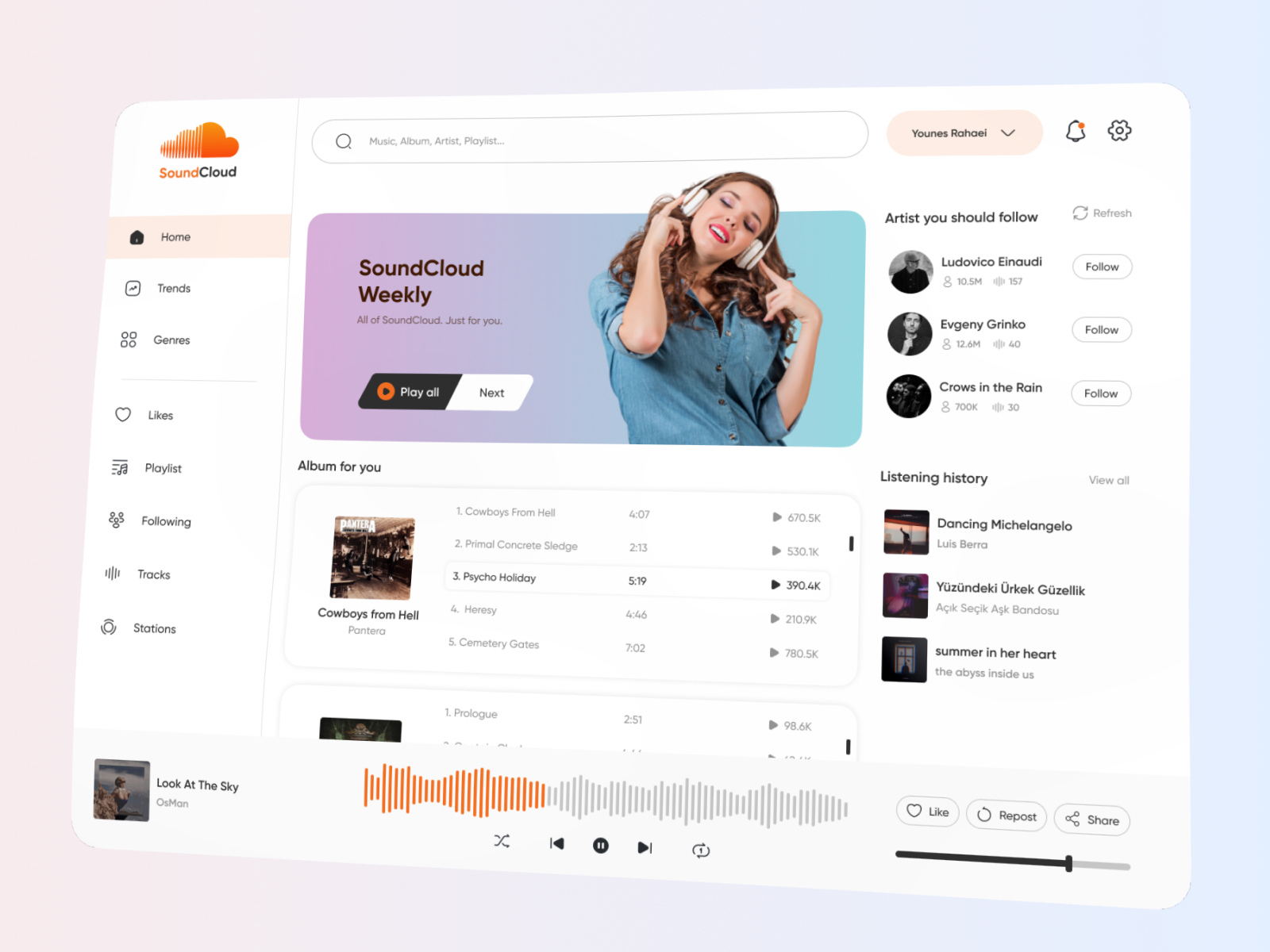The image is a screenshot of a SoundCloud webpage displayed against a pastel background comprising hues of blue, purple, and pink. The webpage is tilted at an angle, slightly skewed, making it difficult to read some of the content clearly. 

At the top of the page, there is the recognizable SoundCloud logo featuring an orange cloud, half of which is solid orange while the other half is striped orange and white. A search bar is present for users to enter information, accompanied by a pink circular icon next to the alerts, and an orange circular icon nearby.

On the left sidebar, there are menu options including categories and playlists, although the angled view makes these labels harder to decipher. 

Central to the webpage is a prominent feature showcasing "SoundCloud Weekly." The section includes an image of a girl wearing a blue button-down shirt and a headset; she is pointing to the headset and has her head cocked slightly. Below this image, there is an option to play the weekly playlist with a 'Next' button. 

Further down, there is a section titled "Album for You," listing what appears to be "Cowboys from Hell" among other tracks. A progress bar indicates that a song from this playlist is almost halfway played, visualized through orange bars.

On the right side of the page, there is a segment entitled "Artists You Should Know," featuring various artist recommendations. Below this, there's a history section displaying recently listened tracks.

Finally, at the bottom of the webpage is a control bar that visually comprises a combination of black and gray segments.